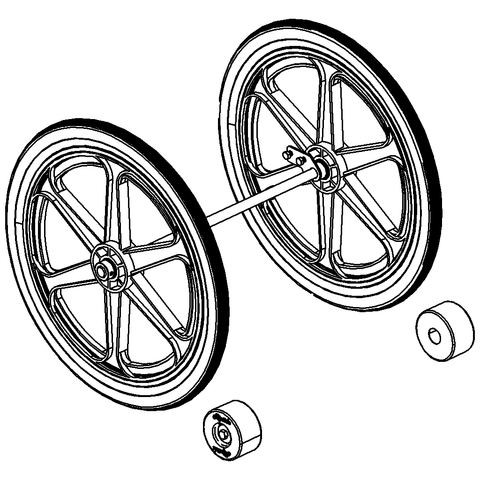The image depicts a detailed black and white diagram of a pair of wagon wheels connected by an axle. Each wheel, located centrally in the composition, features a sophisticated design with six slender, yet distinctly shaped spokes extending from a central hub. The wheels are spaced approximately 1 to 1.25 diameters apart, linked by a meticulously drawn bar or axle running through their centers. Black outlines accentuate the wheels and axle, while the interior areas remain white. Below the wheels, there are two smaller cylindrical objects, each with unique markings. One bears two black lines, while the other resembles a perfect donut. These cylindrical pieces, oriented similarly to the wheels, could suggest bushings or bearings, adding further detail to the engineered appearance of the diagram. The entire illustration floats against a plain white background, without borders, presenting a stark and clear depiction of the mechanical elements.